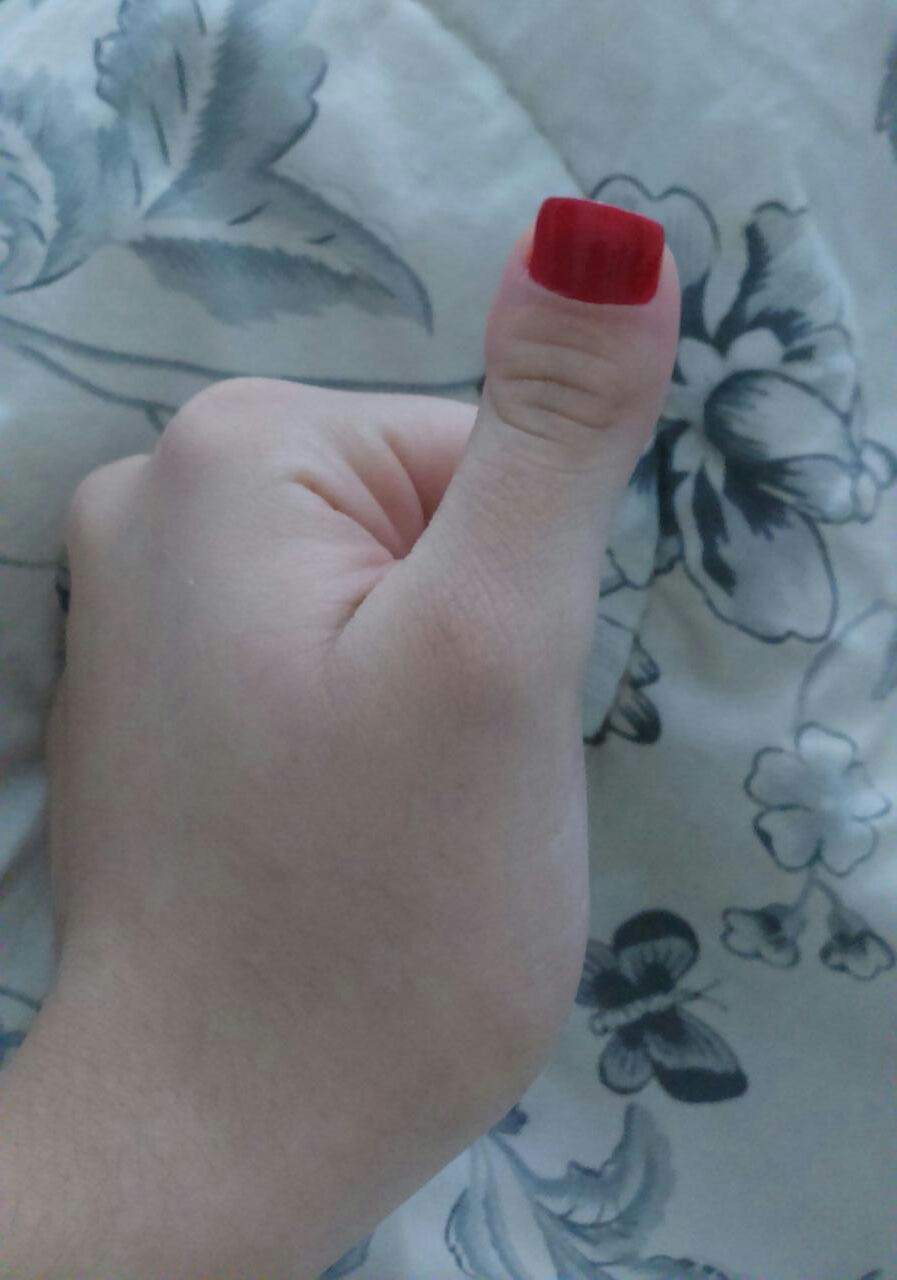This is a close-up, color photograph focusing on a pale-skinned left hand, likely belonging to a young white woman, resting indoors. The hand is clenched in a fist with the thumb conspicuously extended upward. Her thumbnail, featured prominently, appears unusually wide and very short, trimmed to a straight edge that deviates from the typical natural curve. The thumbnail is painted a glossy, deep candy-red color, which starkly contrasts with her smooth, fair complexion. The background consists of a white or off-white blanket adorned with blue flowers, butterflies, and leaves, enhancing the serene indoor setting. The intricate floral pattern appears to be either printed or dyed onto the fabric, adding to the photograph's detailed composition.